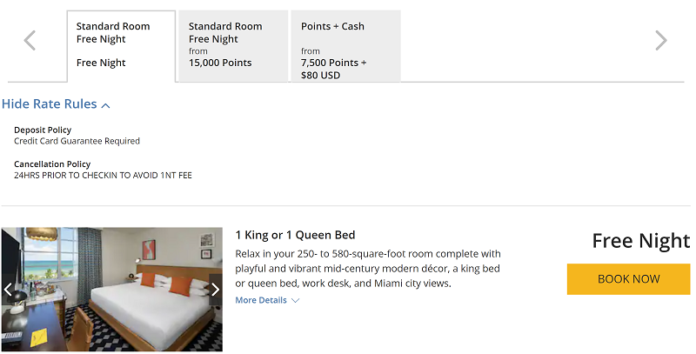This image depicts a hotel booking website. In the upper left-hand corner, there are three distinct tabs for booking options. The first tab is labeled "Standard Room," followed by the text "Free Night." The middle tab, titled "Standard Room," specifies that the free night can be obtained starting from 15,000 points. The final tab is labeled "Points Plus Cash," noting that this option requires a minimum of 7,500 points plus $80 USD.

The "Standard Room" with "Free Night" tab is highlighted in white, indicating it is currently selected. Below these tabs, there is a section that provides details about the room. It includes information that the available room options are either one king or one queen bed. To the right of this text, the phrase "Free Night" is reiterated, and a prominently displayed "Book Now" button invites users to proceed with their reservation.